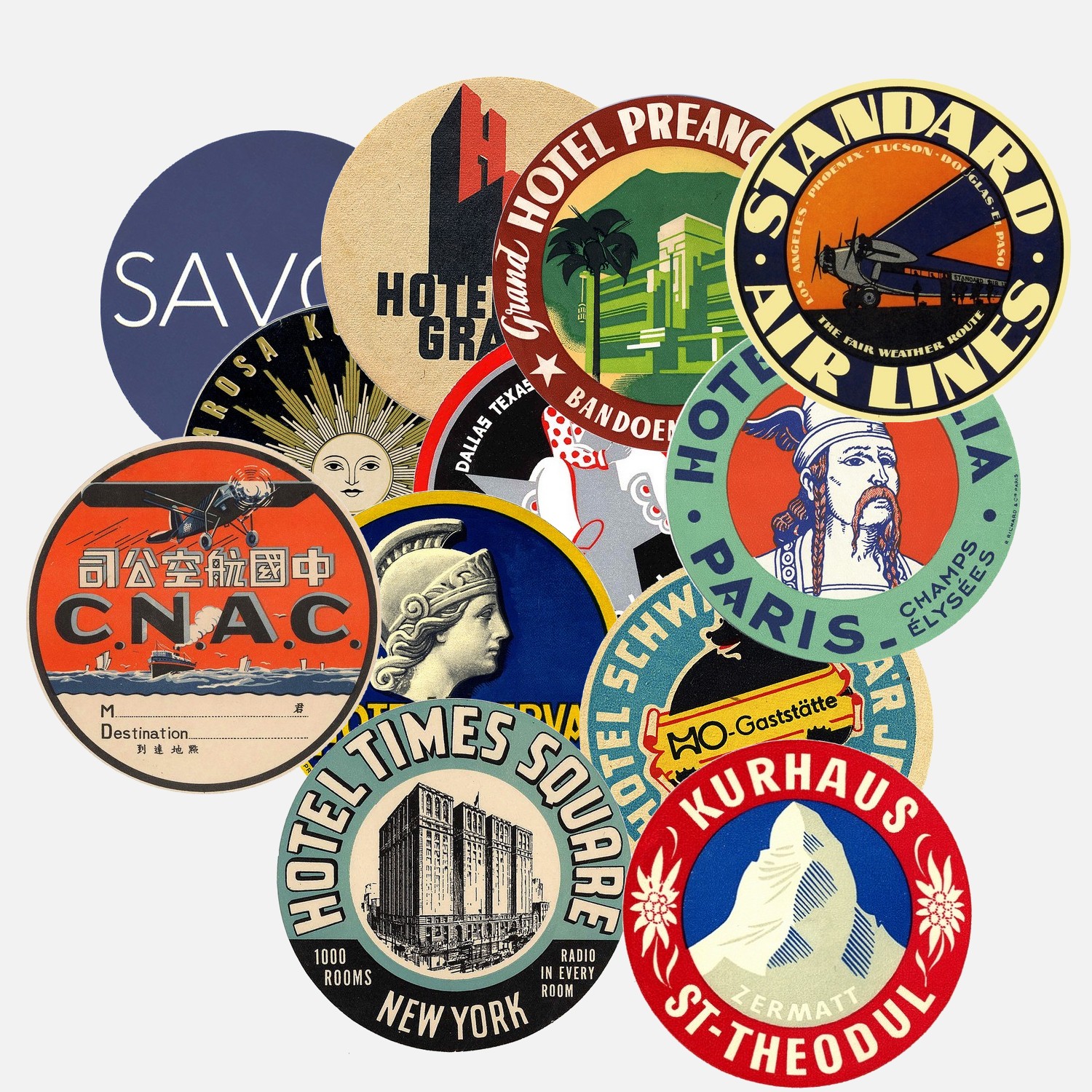The image depicts a vibrant collage of approximately 12 round stickers, logos, or decals, arranged in an overlapping manner. These circular designs come from various places around the world, contributing to an eclectic mix of colors including orange, red, blue, green, and white, all set against an off-white or light gray background. Notable stickers include:

- A "Standard Airlines" sticker in the top right corner, featuring an airplane.
- "Hotel Paris Champs-Elysees" underneath, displaying a figure resembling an oriental man with a long beard.
- A partially visible "Hotel SCHW" sticker with a blue and yellow color scheme.
- "Kurhaus St. Theodol" at the bottom, showcasing a mountain against a blue backdrop.
- "Hotel Times Square" on the bottom left, highlighting “1,000 rooms, New York radio in every room,” accompanied by an illustration of the hotel.
- A red "Zermatt" sticker with a mountain image.
- A sticker with possibly Greek text, situated above the Zermatt one.
- A sticker featuring a Roman warrior.
- Another aviation-themed sticker labeled "CNAC," topped with Chinese characters.
- A "SAV" sticker in solid blue, located at the top left.
- A sunburst design with the label "A-R-O-S-A" and a "K."

Each sticker partially obscures the others, creating a richly detailed montage that suggests global travel and various destinations.